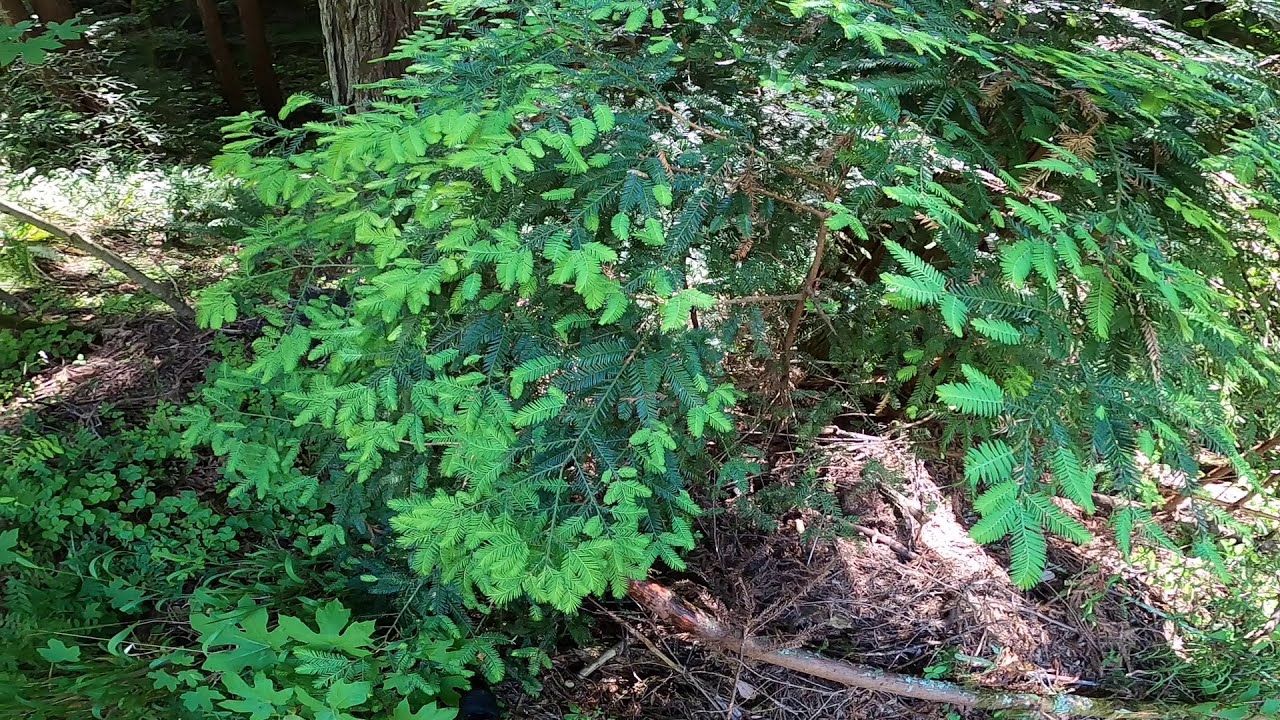The image captures a verdant scene in a rocky, remote woodland, with the focal point being a bush with delicate, slender branches sloping downward. The branches are adorned with long, oval-shaped green leaves that taper to needle-like tips pointing in different directions. The leaves display a gradient of green, lighter on the outside and darker toward the center, where they attach to a light brown stem. Prominently in the foreground, a thick brown stick decorated with green dots crosses from the left and slopes slightly down to the right. In the upper left corner, a dark shadow contrasts with a rough-textured, gray tree trunk, allowing just a hint of sunlight to penetrate. The background reveals an array of branches and twigs strewn across the forest floor, highlighting both the new green growth and the more rugged aspects of the forest. The light indicates daytime, illuminating the plant and accentuating various textures and colors.